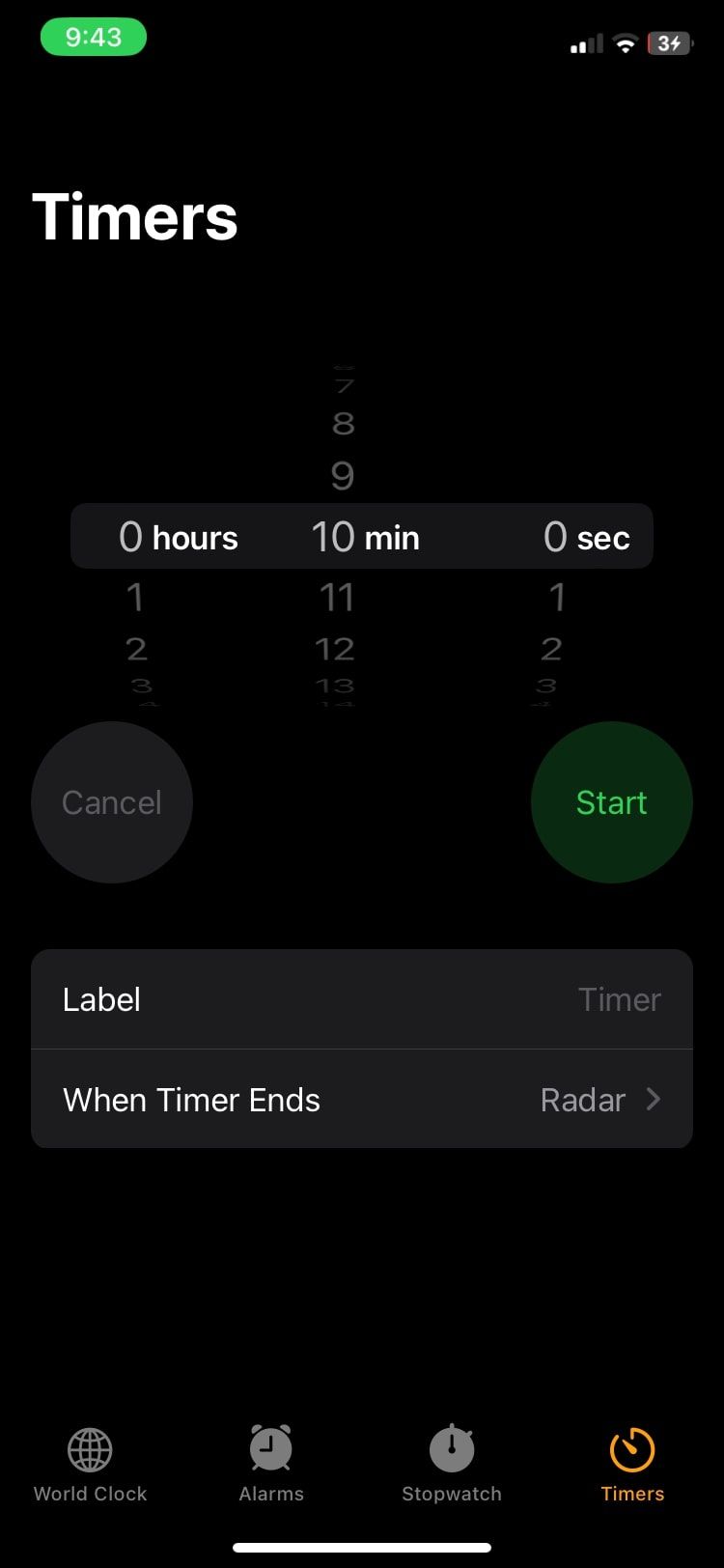This image is a screenshot from a smartphone. The background is completely black. At the top of the screen, on the left, there is a small green oval displaying the time "9:43 AM" in white text. On the right side of this bar, there are icons indicating the Wi-Fi signal, cell phone signal strength, and battery percentage, which shows a lightning bolt symbol next to it, suggesting the phone is currently charging.

Beneath this, on the left side of the screen in a larger font, the word "Timers" is prominently displayed with a capital "T". Below this header, the current timer reads "0 hours 10 minutes 0 sec," and each of these units (hours, minutes, seconds) is accompanied by a faintly visible sequence of numbers indicating an incrementally increasing count: under the "hours," the numbers "1, 2," and a partial "3" can be seen faintly; under the "minutes," the sequence "8, 9, 10" is visible with "10" in bold, followed by lighter "11" and "12" markers; and under the "seconds," the sequence "1, 2," and part of a "3" is visible.

At the bottom of this timer display, there is a grey circular button labeled "Cancel". Next to it, there is another circular button, which is tinted a darker green, with a brighter green label that reads "Start" indicating the action button for starting the timer. Under the label, it says “When Timer Ends: Radar.”

At the very bottom of the screen, there are tabs for different functions. These include "World Clock," "Alarm," "Stopwatch," and "Timers," indicating different features of the clock application.